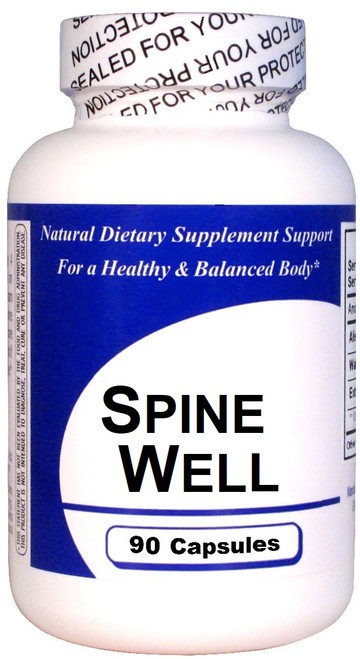This image features a close-up of a supplement bottle, occupying almost the entire frame. The background is a plain white, emphasizing the product itself, which is a standard white plastic pill bottle with an opaque surface, preventing any view of its contents. The bottle's white cap is slightly narrower than the bottle and is sealed with a clear plastic safety seal that displays the text "Sealed for your protection" in black letters, arranged diagonally.

The bottle's label is designed with a combination of black, white, and blue colors. At the top of the label, the text reads "Natural Dietary Supplement Support for a Healthy and Balanced Body" in white letters against a bright, sky-blue background, featuring a small asterisk. Below this, the label transitions to a white area where "Spine Well" is printed, followed by a blue horizontal line, and then the text "90 capsules" within a small rectangular box. Slightly visible on the label's left and right edges are partial glimpses of additional information, such as a nutritional label and possible warning or usage instructions, though they are not fully legible due to the front-facing view of the bottle.

Overall, the image resembles a typical product shot intended for an e-commerce website, highlighting the supplement's branding and essential details clearly.